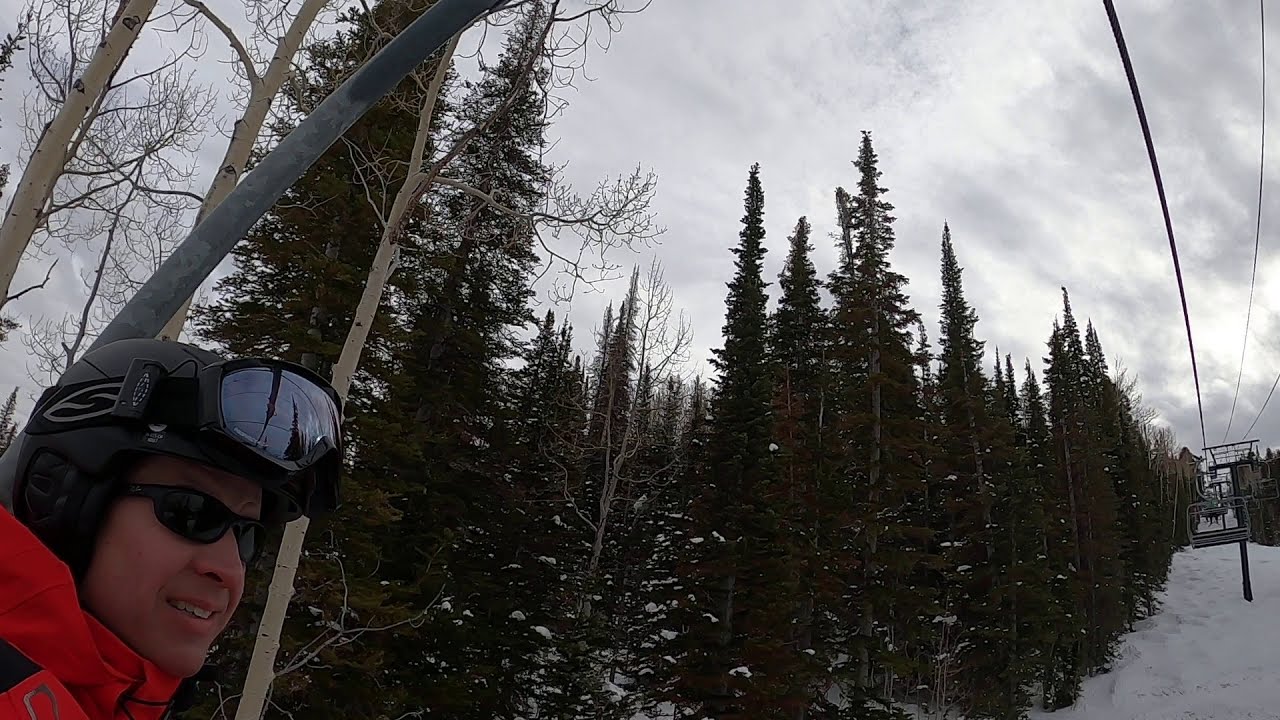In this detailed image of a winter scene at a ski resort, a man in a reddish-orange ski jacket and black ski cap is prominently featured in the bottom left corner. He is smiling broadly, revealing his teeth beneath his sunglasses, while his ski goggles rest atop his cap. The ground is blanketed with snow, and to the right, a ski lift stretches into the distance, its gondolas suspended silently from the cables. Tall, thin trees, covered lightly with snow, frame the left side of the scene, consisting of a mix of evergreens and deciduous trees, potentially birches. The sky is overcast and gray, indicating a cold winter day with no visible sunshine. This serene and chilly outdoor setting captures the essence of a quiet day on the slopes.